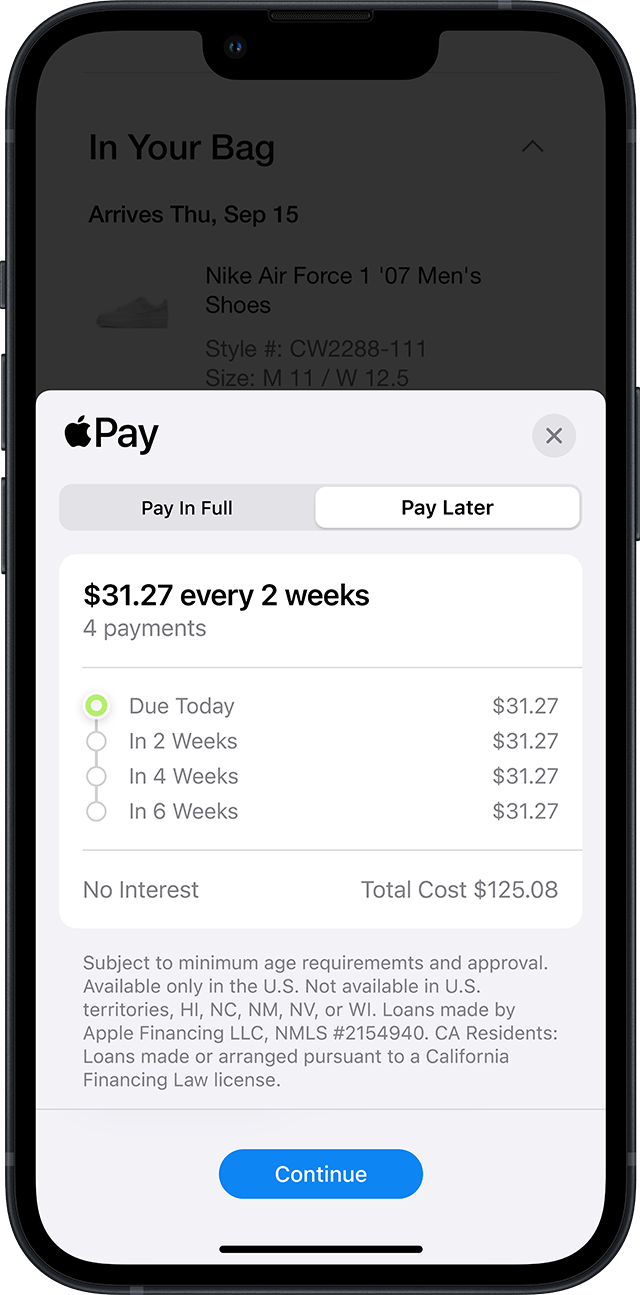The image depicts a vertical smartphone screen, approximately 2.5 to 3 times taller than it is wide. The device is framed by a black border, with the camera and speaker visibly positioned horizontally at the top. The screen is active, displaying an Apple Pay interface.

In the upper left corner, a black Apple logo is accompanied by the word "Pay." On the upper right, an 'X' icon is present for closing the interface. Below this, two horizontally aligned option buttons are visible: "Pay in Full" (grayed out) on the left and "Pay Later" (highlighted in white) on the right, indicating the latter is selected.

The main content area of the screen, occupying roughly two-thirds of the display from the bottom, features a title in bold black text: "$31.27 every two weeks." Beneath this, in gray text, the phrase "for payments" is noted. Four options are listed in bubble format, with the first bubble highlighted in green and marked "Due today." The subsequent bubbles are labeled "In two weeks," "In four weeks," and "In six weeks," respectively, and remain unselected.